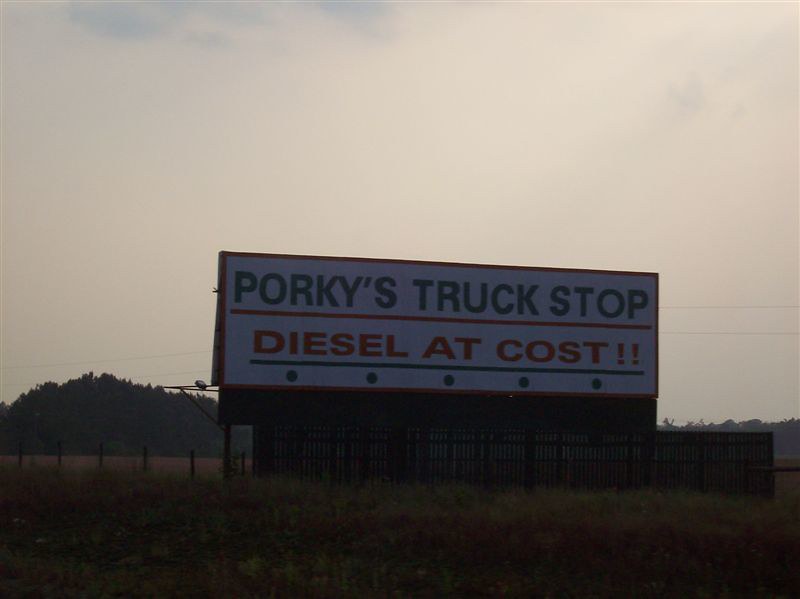A photograph captures a rustic billboard set in a tranquil countryside landscape. The billboard, which stands approximately four to five feet off the ground, is enclosed by a modest metal fence supported by several small fence posts. The foreground features a mix of grass and dirt, adding to the rural ambiance. In the background, a series of densely vegetated hills or mountains rise, providing a lush, green contrast to the scene.

The billboard itself is primarily white and prominently displays its message in bold, colorful text. At the top, light blue, all-capital letters spell out "Porky's Truck Stop," accentuated by an orange underline. Below this, in striking orange text also underlined, but in the same light blue, the sign reads "Diesel at Cost."

This succinct yet vivid advertisement suggests that Porky's Truck Stop offers diesel fuel at cost price, making it an attractive stop for travelers in this serene, country locale.